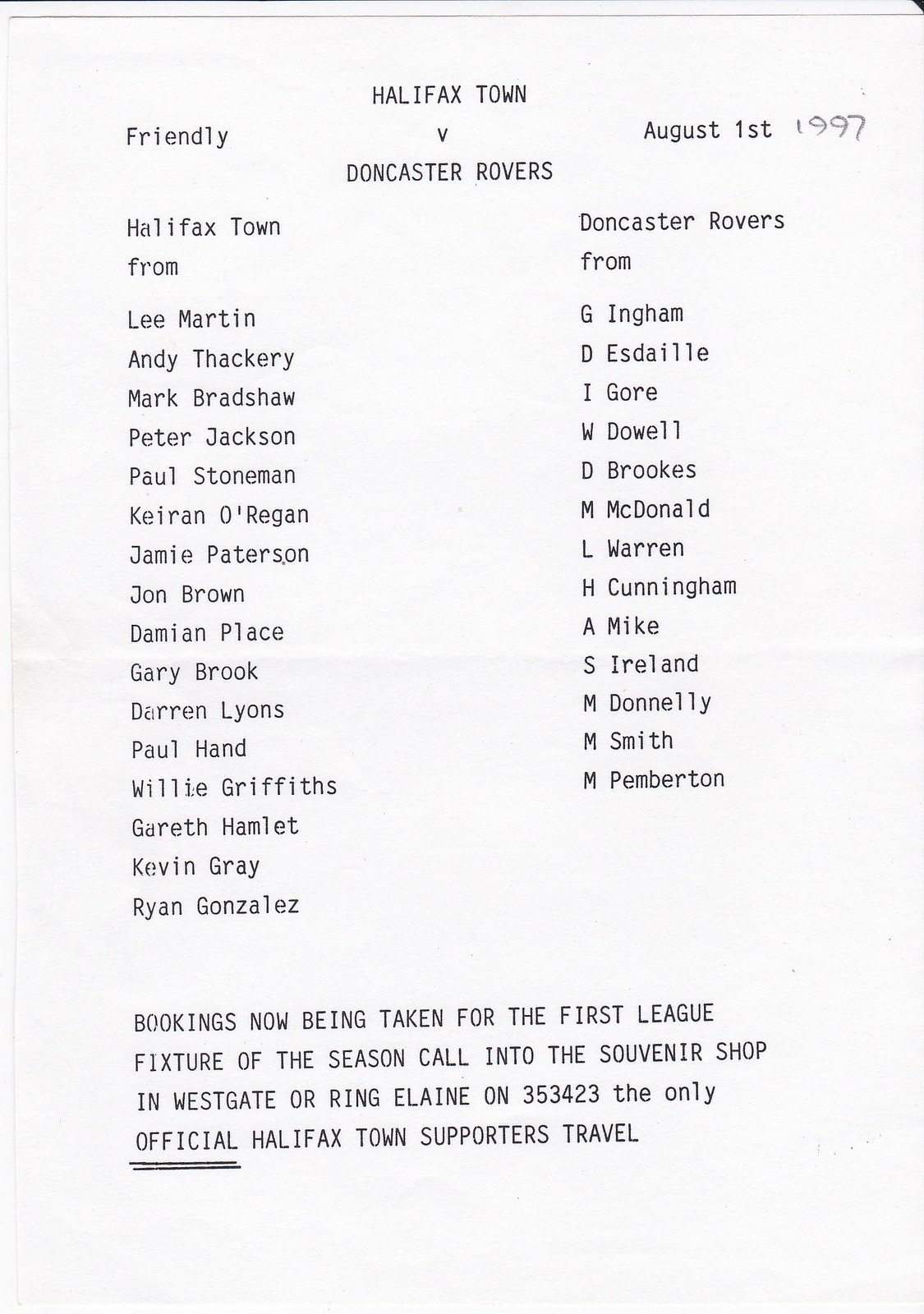The image captures a scanned poster from a 1997 sports program advertising a friendly soccer match between Halifax Town and Doncaster Rovers. The top of the page prominently features "Halifax Town vs. Doncaster Rovers" followed by the date "August 1st, 1997" with "Friendly" marked in the upper left corner. The poster is organized into two main columns: the left column starts with "Halifax Town from" and lists players including Lee Martin, Andy Thackeray, Mark Bradshaw, Peter Jackson, and Paul Snowman. The right column begins with "Doncaster Rovers from" and lists players by their initials and last names, such as G. Ingham, D. S. Daly, I. Gore, W. Dowell, and D. Brooks. At the bottom of the page, there's a promotional paragraph stating, "Bookings now being taken for the first league fixture of the season. Call into the souvenir shop in Westgate or ring Elaine at 353-423, the only official Halifax Town supporters travel." The document appears primarily in black and white and takes up the entirety of the image, serving as an advertisement for both the match and a souvenir shop.